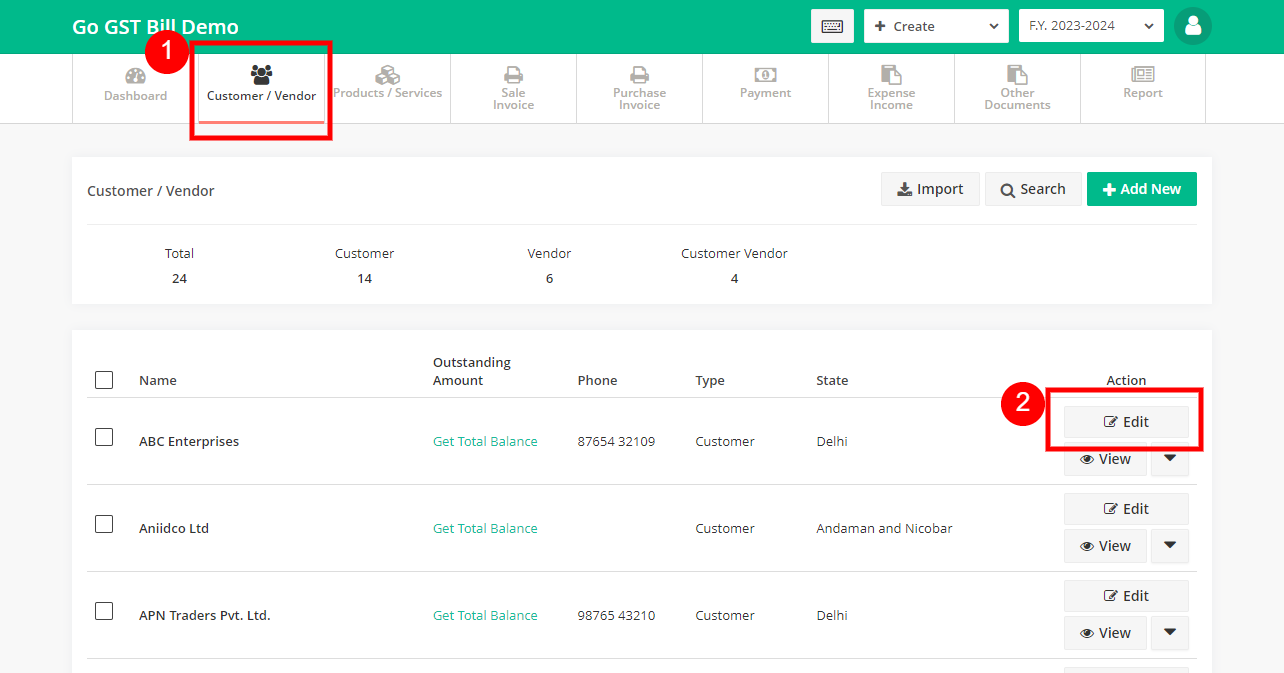This cropped screenshot showcases a horizontally oriented PC application interface, implying a desktop environment. The top menu banner features a green background with white text that reads "Go GST Build Demo." Adjacent to this text, on the right side, there is a small grey icon within a square, though its details are indistinguishable at this resolution. 

To the right of the icon, a white drop-down menu with a plus symbol marked "Create" offers additional options when clicked. Next to it, another drop-down menu is labeled "FY 2023-2024," indicating the selected fiscal year. Near the far right, an icon resembling a person, likely denotes the user profile button.

Below the menu banner, there is a vertical list of icons each accompanied by labels, primarily depicted in black or grey. The icons indicate different sections: Dashboard, Customer/Vendor, Product/Services, Sales Invoice, Purchase Invoice, Payment, Expense, and Other Documents. Notably, the icon for "Customer/Vendor" is selected and highlighted with a red box marked by the number "1." This suggests it is the currently active section.

In the bottom-right corner, there is a table or list characterized by check marks and columns. The last column is titled "Action," featuring an "Edit" button. This button is also highlighted with a red box labeled with the number "2," indicating its importance or to draw attention to it.